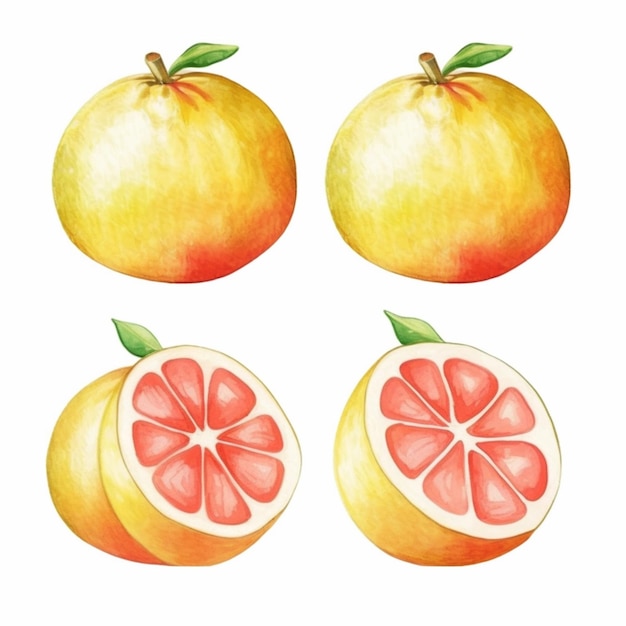This is a detailed drawing or painting of four grapefruit against a white background, arranged in two rows. In the top row, there are two whole grapefruits, each with a yellowish-orange hue and a hint of red at the bottom. Both fruits have a stem with a single leaf extending from it. The bottom row features two halved grapefruits, revealing their interior segments. Each half displays eight segments surrounded by the white pith, with the flesh exhibiting a peachish-pink color. Notably, the fruit in the lower left appears to have an unusual, two-part structure, resembling two connected lobes with one lobe sliced open. Each cut fruit also has a leaf extending from the top, mirroring the arrangement of the whole fruits above. The meticulous attention to detail in the painting highlights the texture and color variations within the fruit, emphasizing its resemblance to grapefruit.